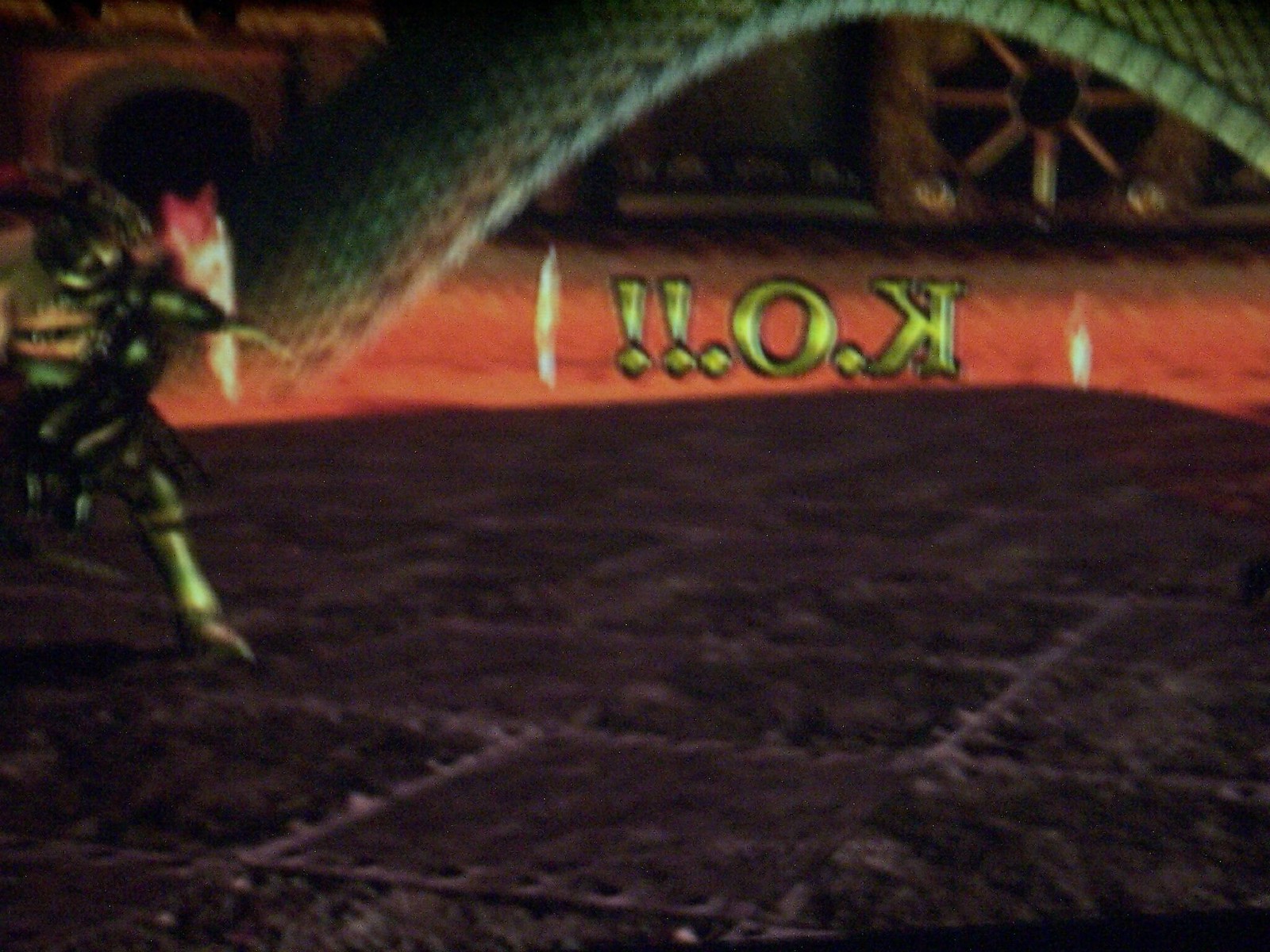This image showcases a rich, deeply colored Persian rug featuring a rectangular design with intricate patterns in deep red and white hues. Lying above the carpet is an elongated piece of red fabric or tube, adorned with a green arch. Bold white letters are emblazoned across the red section, displaying an unusual sequence: two exclamation marks, followed by a period, an 'O', another period, and a reversed 'K'. Several vertical white lines run parallel on this red item. In the background, to the right, a spoked wooden wheel can be discerned, accompanied by partially visible objects that contribute to the intricate setting of the scene.